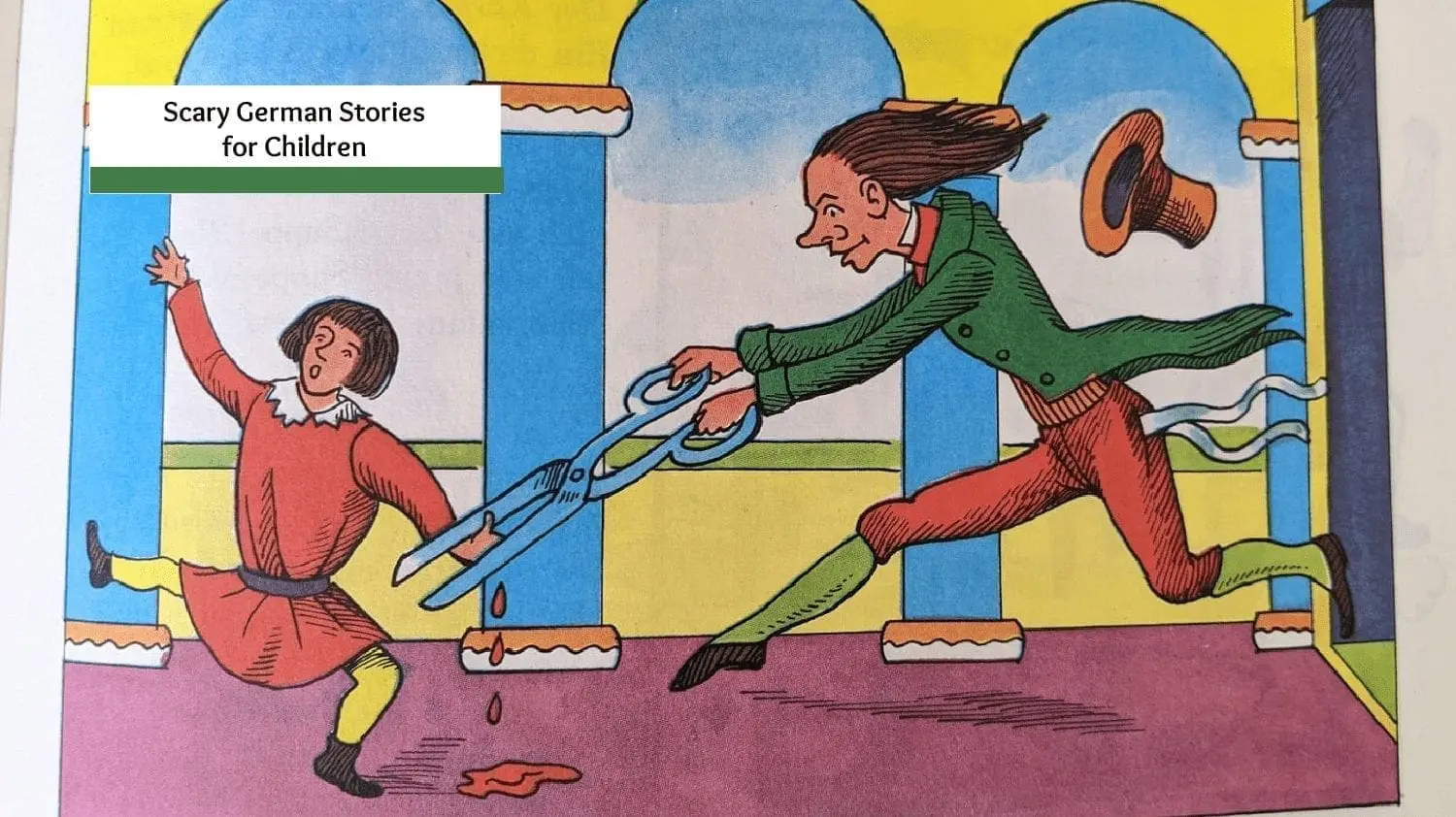This image, resembling a comic panel from a book, depicts a vividly colorful yet grim scene titled "Scary German Stories for Children." The caption is presented in black text within a white box, offset by a green border, positioned in the top left corner. The cartoon features a young child with brown hair, dressed in a red dress and yellow pants, standing precariously on one leg with an alarmed expression as their right hand or fingers are being cut by a giant pair of scissors. Blood drips down from the injury. The child raises one arm while the other arm is clamped by the scissors.

A sinister man, seemingly enjoying the act, prances or jumps toward the child. He has long brown hair, wears a vibrant green jacket, orange or red knee-length pants, green socks, and large shoes. His top hat has flown off his head amidst the commotion. The background is strikingly colorful, featuring yellow walls, green pillars, and a purple ground, with three arches framing a gradient sky of blue, white, and yellow hues. The overall scene is detailed and grotesque, fitting the eerie title of "Scary German Stories for Children."